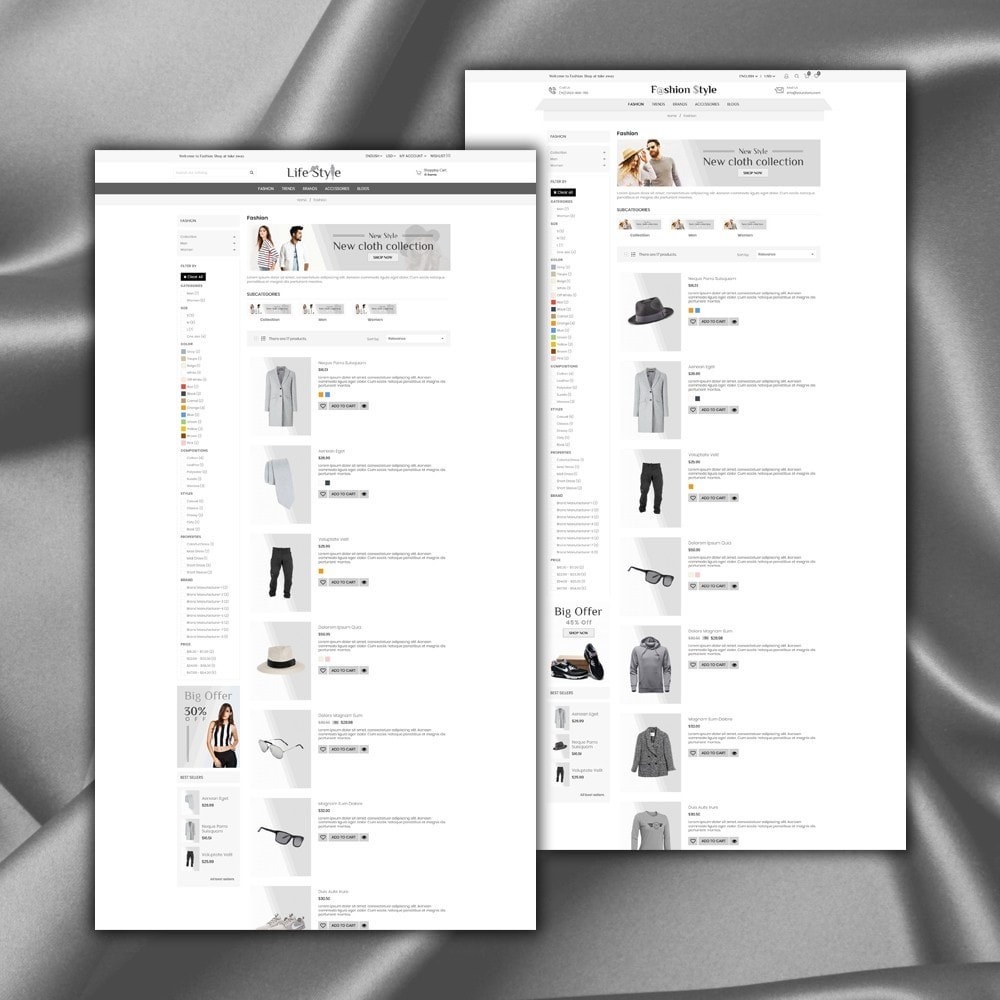In this image, we observe two nearly identical websites side by side, with one slightly overlapping the other to the left, obscuring a small portion. Both websites are dedicated to showcasing clothing collections. The background appears to be a silver, rippled material that resembles folded metallic fabric, adding an interesting texture to the overall visual.

The first website on the left features a dark gray banner with "Lifestyle" written on it and promotes a "New Cloth Collection." The displayed items include a long jacket, a tie, gray pants, a white hat with a black headband, sunglasses, and sneakers, arranged neatly to highlight the variety in the collection.

The second website on the right shares a strikingly similar design but is branded as "Fashion Style" at the top. It also advertises a "New Style New Cloth Collection," displaying comparable items. Within this collection, you'll find a darker gray hat, a hoodie, and several jackets, indicating slight variations in the offerings between the two platforms.

Together, these websites demonstrate a cohesive fashion theme, with minor differences in the presented clothing items, reflecting similar yet distinct brands.